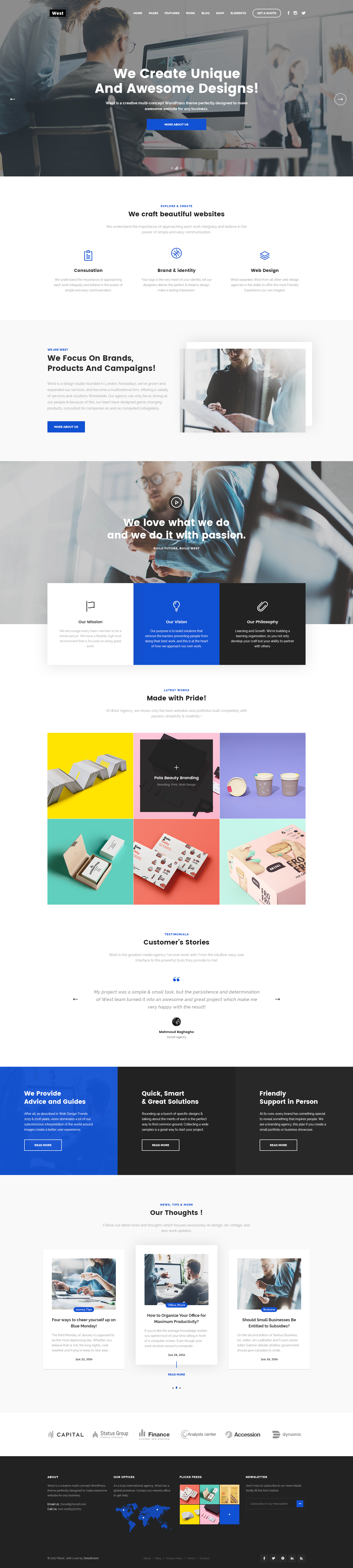The image depicts a vertically stretched website, making it difficult to read text without significant enlargement. At the top left corner of the page, a button labeled “West” is followed by navigation options in a horizontal line: Home, Pages, Features, Work, Blog, Shop, Elements, and Get a Quote. Additionally, icons for Facebook, Instagram, and Twitter are present.

Beneath the navigation bar, there is a prominent header in large font stating, "We Create Unique and Awesome Designs!" This is followed by a description of "West," a creative multi-concept WordPress theme designed to build impressive websites for any business, with a prompt to "See more about us."

Further down, sections with headings like "Explore and Create" and "We craft beautiful websites" emphasize the importance of integrating each project and maintaining simple communication. Another section titled "Brand and Identity" highlights the significance of a logo in defining one’s identity, boasting that their designers can deliver perfect and memorable designs, though the distorted layout makes this text challenging to read.